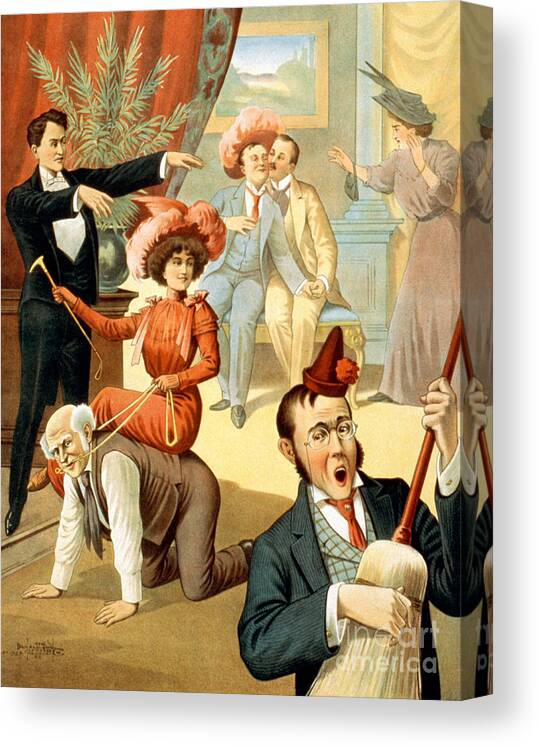This canvas print, titled "Fine Art America," depicts a whimsical, vintage party scene reminiscent of a setting from the Clue board game. In the foreground, a man with spectacles and a receding hairline, wearing a red cone hat adorned with a puff, is playfully performing with a broom as if it were a guitar, his mouth wide open in mid-song. His attire includes a three-piece suit, adding to the jovial atmosphere.

Behind him, a heavy, ornate red velvet curtain is drawn to the left, revealing a lively background. A woman in a big gray hat and a powder pink dress, appearing shocked and slightly rushing in, reaches towards two men. One man is in a dark blue tuxedo with a red tie, kissing another man on the cheek who is in a lighter, camel-colored suit. This affectionate moment contrasts with the chaotic energy surrounding them.

To the foreground's left, a woman dressed in an orange outfit complete with a matching hat holds a whip and has a leash around the neck of a kneeling balding man in tan pants and a vest. Her dominant pose adds another layer of eccentricity to the scene. A large plant positioned behind a tuxedo-wearing man with outstretched arms, resembling a zombie, completes this eclectic portrayal, embodying a blend of vaudevillian, 1800s, and Victorian-era influences. The overall image exudes a sense of playful chaos, capturing an era of vintage revelry with a whimsical twist.